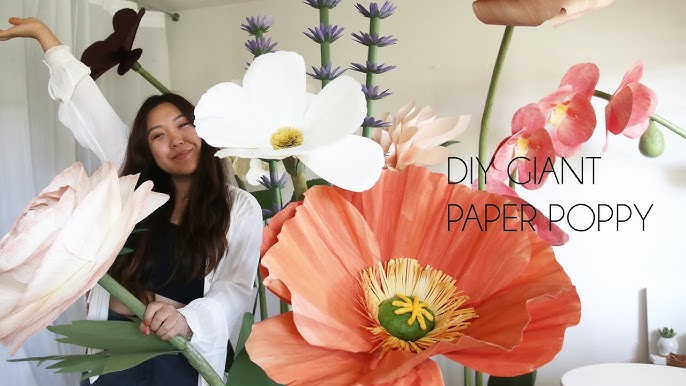The image features an Asian woman with long dark hair and tan skin, smiling gently without showing her teeth. She is dressed in a dark-colored shirt paired with a white over-jacket. She stands against a backdrop of giant, intricately crafted paper poppies in vibrant hues of white, peach, orange, and light pink. The flowers, some featuring yellow interiors and green buttons, are adorned with a sans-serif text that reads "DIY Giant Paper Poppy." The setting appears to be a well-lit room with white curtains, white walls, and a lamp accentuating the beauty of her paper creations. The composition highlights the woman’s evident joy and pride in her artistic hobby of making enormous, realistic paper flowers.